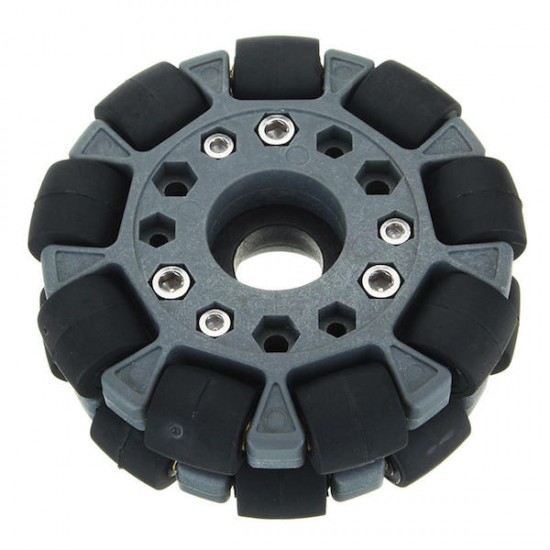The photograph showcases a mechanical assembly consisting of two circular gray objects, possibly made of metal and plastic, stacked vertically on top of one another. Each circle features a central cutout, resembling a wheel shape, potentially designed for a pole or post to pass through. The objects are interconnected by six metal screws that traverse hexagon-shaped cutouts, securing the two circles together. Around the outer edges of the circles are multiple small black wheels arranged vertically, running counter to the circular shape. Some of these wheels are visible on a second, partially obscured layer beneath the main assembly. The contrasting gray and black components stand out sharply against the plain white background, emphasizing the detailed structure and components of the object.